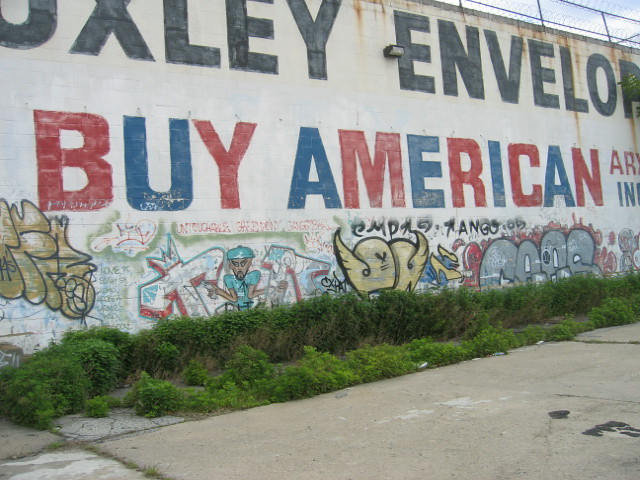The image captures the exterior of a building with a tall, predominantly white wall, adorned with various writings and graffiti. At the top of the wall, in black lettering, it reads "Oxley Envelope." Below this, in alternating red and blue letters, it says "Buy American." Further down, there's a vibrant array of graffiti including brown bubble-style letters, red and blue crosses, random objects, and an illustrated elephant with discernible ears and face. Among the graffiti, a small figure can be seen, dressed in blue clothing and a blue cap, sporting a mustache and a small beard, seemingly holding paint cans. Directly in front of the wall, there are small shrubs and concrete paving. The top of the wall features a barbed wire fence, adding to the urban aesthetic.